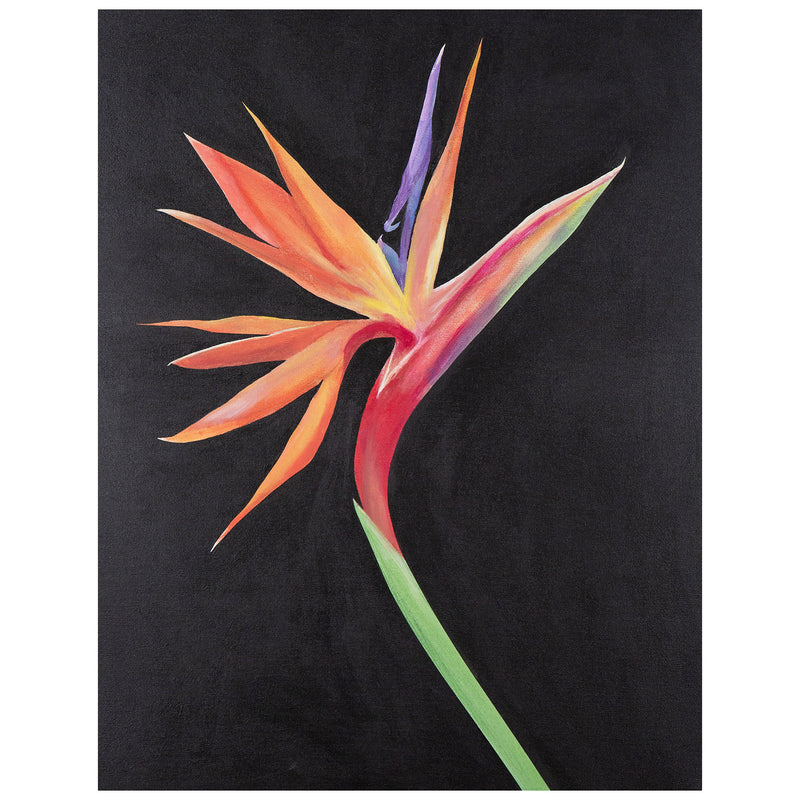The image is a vertically oriented, abstract drawing of a Bird of Paradise flower set against a completely black background. The flower’s vivid coloring includes red, orange, yellow, green, and a distinctively prominent purple petal. The stem starts in the lower right-hand corner, climbing diagonally towards the middle of the frame before curving upward. The flower head occupies the central portion of the image, with its pointy petals radiating outwards, some extending almost to the top. The petals vary in color; most are orange or yellowish-orange, with a particularly striking purple petal at the center, accented with a blue hue and a reverse barb. One petal transitions from red at the base to green at the tip. The black backdrop accentuates the bright, vivid colors, though the image is not very sharp and no other elements are present.